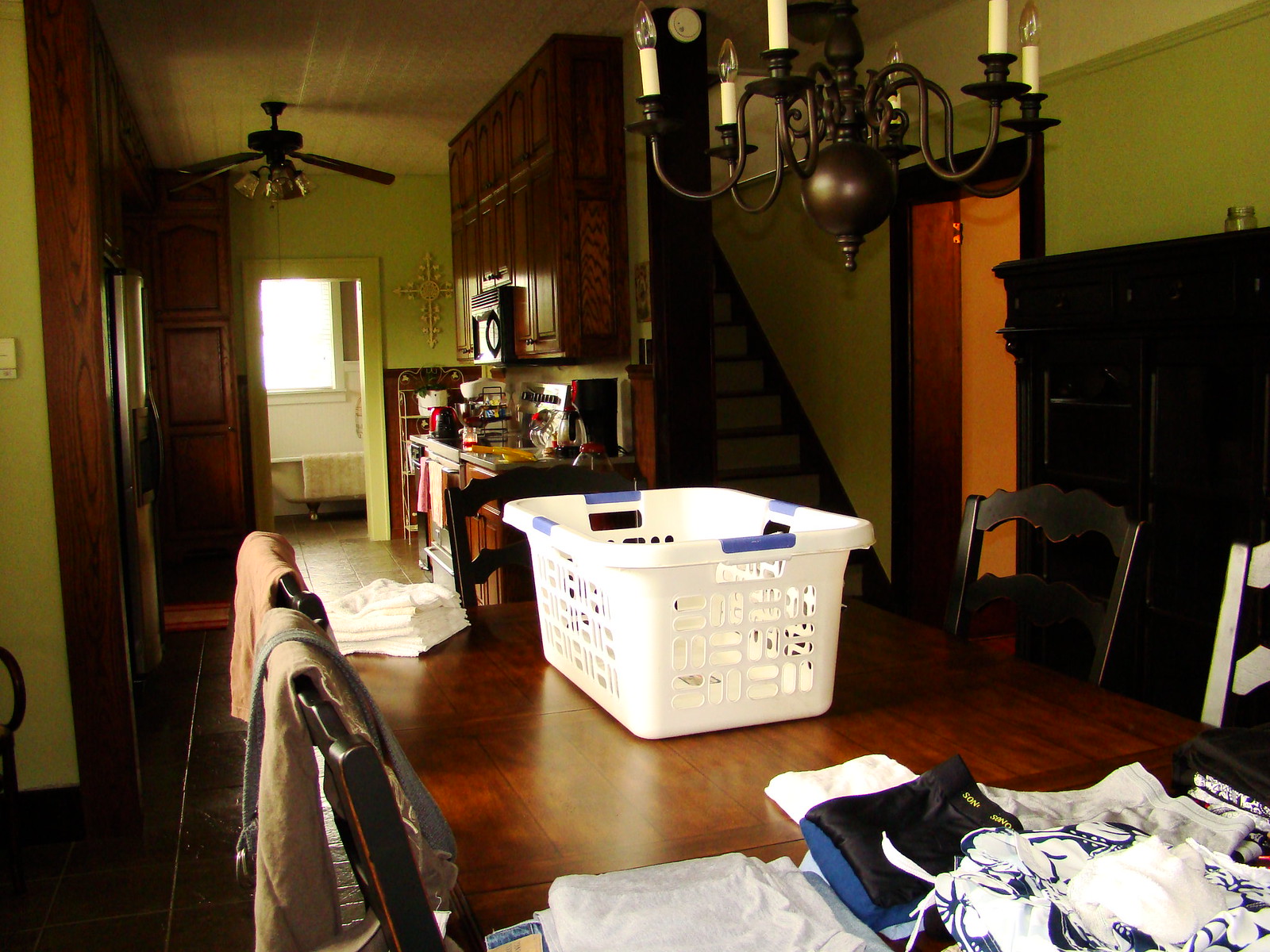The image showcases the cozy interior of a home, drawing attention to a polished, deep brown wooden dining table set centrally in the room. The table is surrounded by five matching wooden chairs, each gracefully crafted to complement the robust design. Atop the table rests a pristine white, rectangular laundry basket filled with neatly folded clothes, indicating a moment of domestic tidiness. Some garments are casually draped over two chairs on the left, adding a lived-in feel to the scene. Suspended above the dining table, a chandelier of deep burnished copper emits a warm, inviting glow, enhancing the homey atmosphere.

In the background, a hallway extends further into the home, leading to a kitchen area visible with cabinets and countertops cluttered with everyday items, reflecting the active life within the household. To the right, a stairway ascends to the upper floor, next to which stands a sturdy wooden cabinet, snugly positioned against the wall. The overall scene captures a snapshot of everyday life, blending functionality with the comfort of a well-loved home.